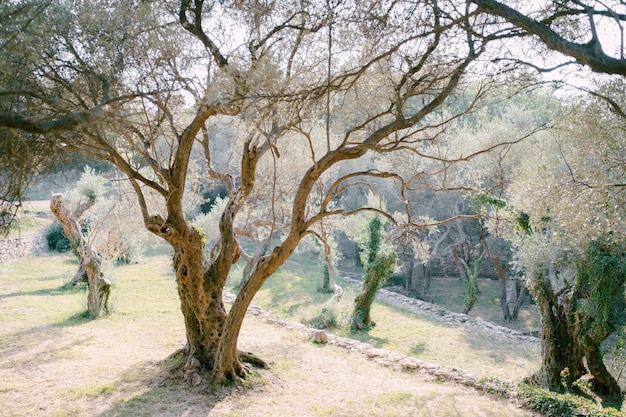The image is a rectangular painting, wider than it is tall, depicting a serene and mystical garden. Dominating the scene, just left of center, is a large, old tree with a sprawling trunk that branches out in multiple directions. The tree is primarily bare, with sparse green leaves and white blossoms near the top sections of its branches. It also features numerous holes in its aged trunk. 

Surrounding the central tree is a light-colored grassy patch, accented with green hues. The garden extends into the background with a variety of other trees, creating a layered effect that resembles steps. Towards the background on the right, a thick tree trunk and smaller trees are visible amidst the greenery.

The overall scene radiates tranquility with its soft lighting and the white sky above, enhancing the mystical atmosphere. In the faint background, there's a small brick wall, adding a touch of structure to this enchanting outdoor space.